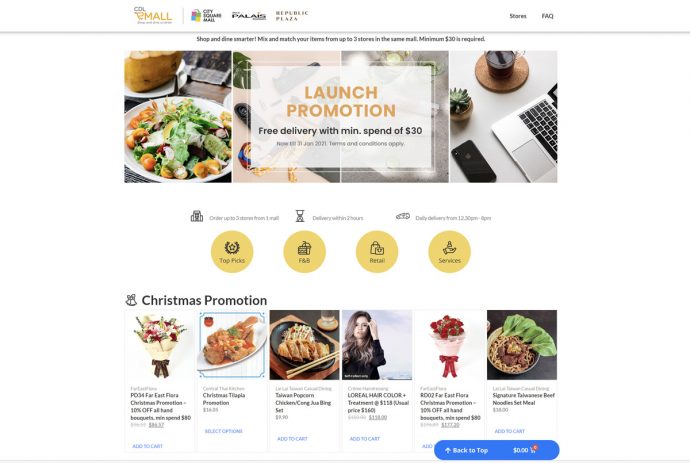The image depicts a screenshot of a web page, presumably related to food. At the top, there is a small, somewhat indistinguishable yellow text, possibly saying "small" or "mall," accompanied by a light gray line. The header features a row of four pictures. A white box obscures the center two images, containing text that announces a "Launch Promotion: Free delivery with a minimum spend of $30."

To the left of this box is a clear image of a large plate of salad. On the right, there is a scene with a laptop, a cup (potentially filled with coffee or juice), and a small succulent plant beside it. Below these images, there are four yellow circles, each containing different words and icons. Above these circles, three additional black icons are displayed on a white background.

Further down, the web page advertises a "Christmas Promotion," displaying six square images in a row. Each of these images has descriptive text beneath them. While most images show various types of food, the center picture features a woman. The bottom right two images are partially covered by a blue, rounded rectangle shape.